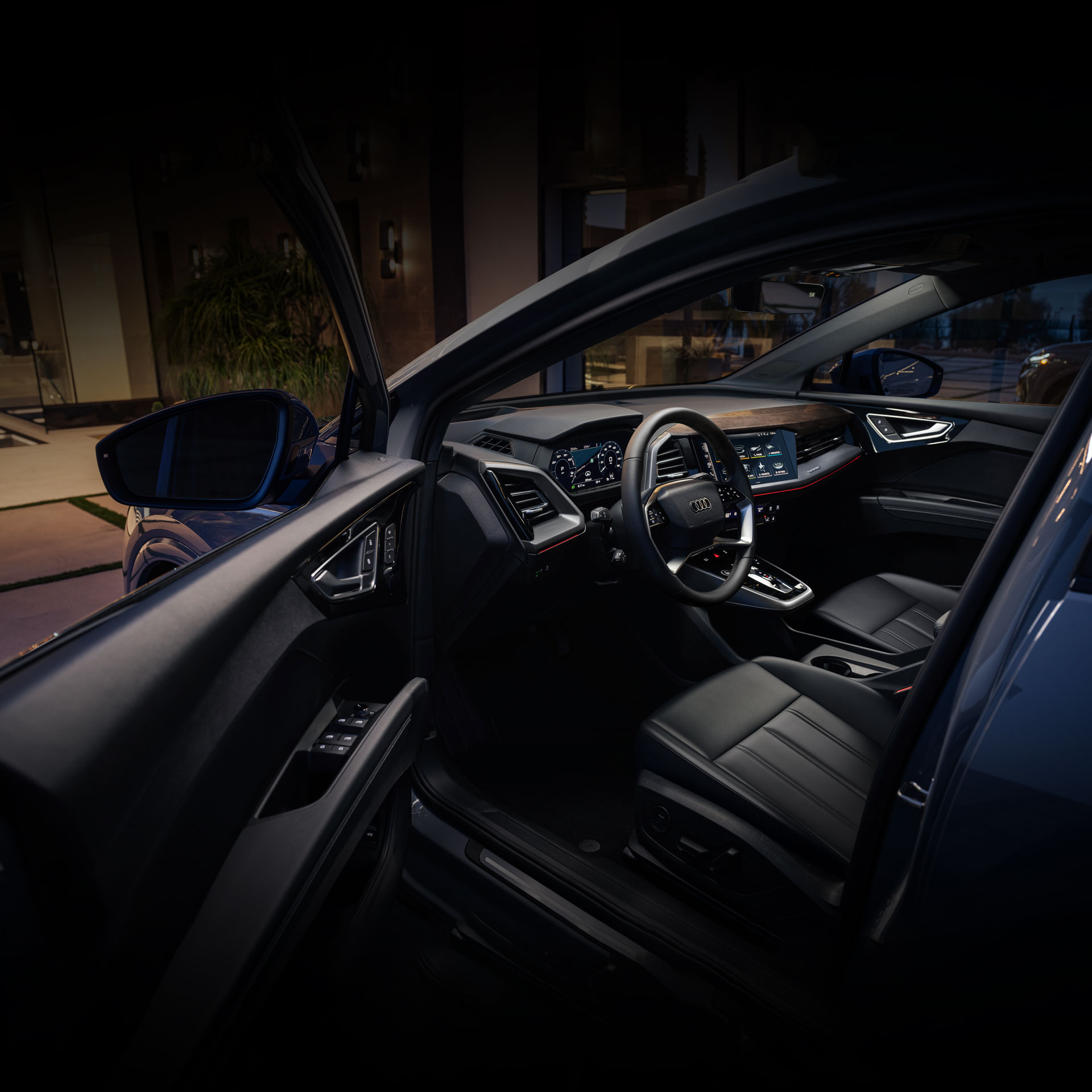The image depicts a dimly-lit interior of a dark-colored Audi car, with the driver's side door open, suggesting it's parked in a garage or high-end area, possibly near a sidewalk with storefronts or a sophisticated building with glass exteriors. The angle is from outside the vehicle, focusing on the luxurious black interior with the steering wheel, dashboard gauges, and screens all illuminated, highlighting the refined leather seats and sleek controls on the armrest and door, including window and lock buttons. The interior lighting and vignette effect cast a professional ambiance, ensuring no harsh reflections and emphasizing the cleanliness of the car's components.